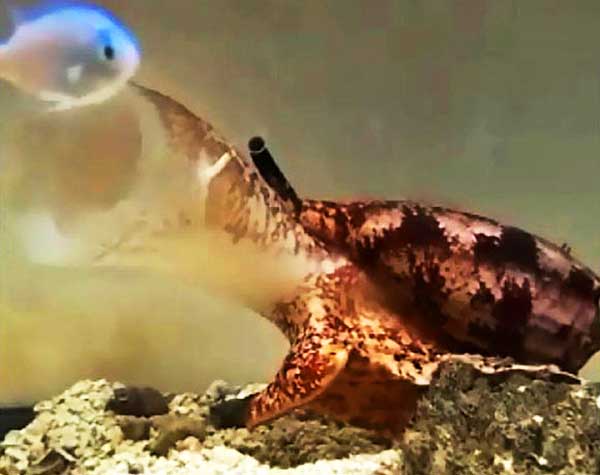This underwater photograph, likely taken in an aquarium, features a small, indeterminate creature that could be a salamander or perhaps another type of aquatic animal. The creature is predominantly orange, red, and pink in color, with speckled black and white areas. It has an open mouth aimed towards the top left corner of the image where a blurred, white fish with pink hues and blue outlines or fins is partially visible. The creature's head is amidst a cloudy, murky part of the water, adding to the overall blur and making identification challenging. The creature is positioned on a bed of light brown and tan rocks, and a distinct stone is visible at the bottom right of the image. The background of the photograph is also quite murky, especially towards the left, suggesting stirred-up sand or sediment.